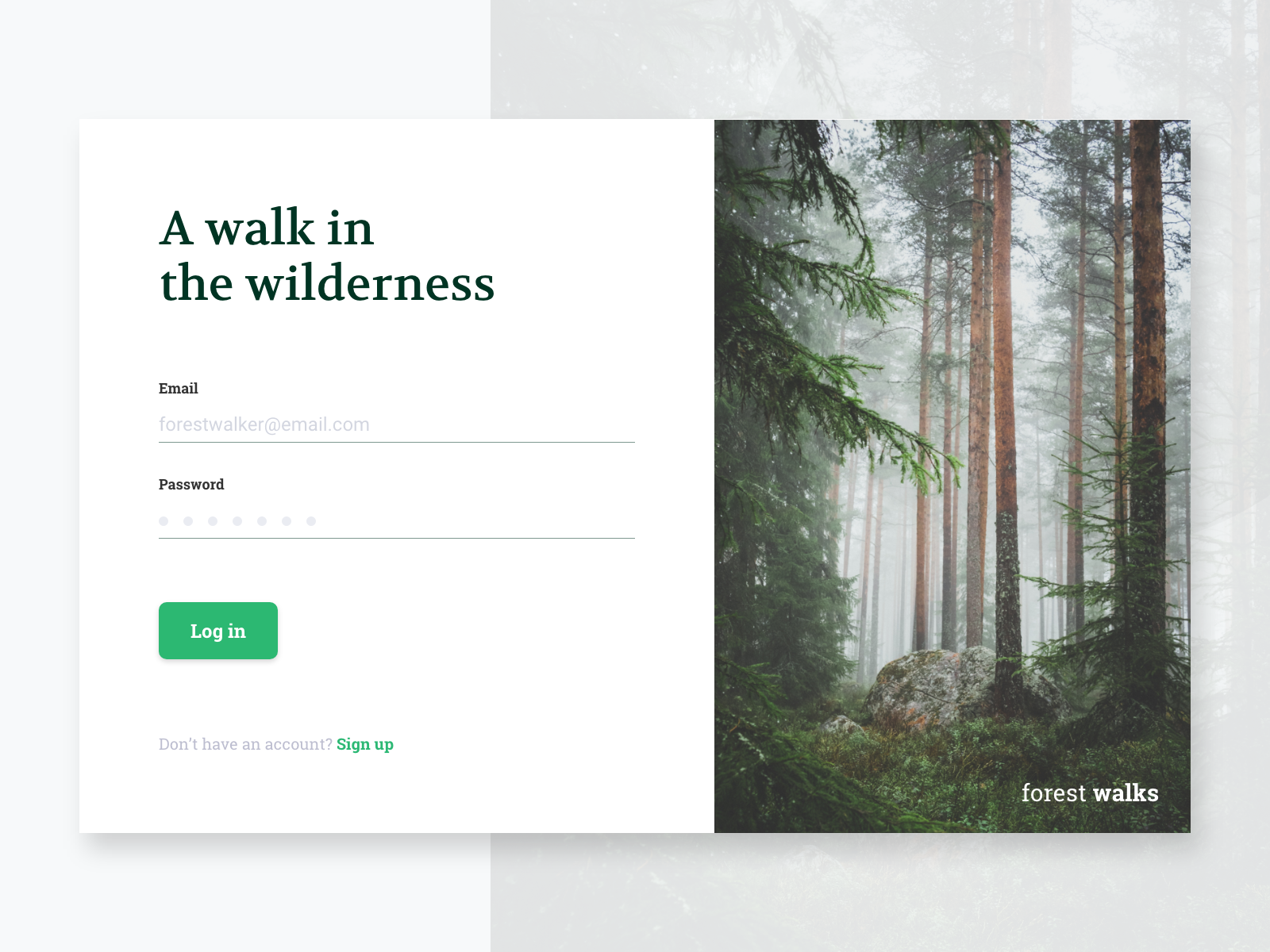This image showcases a screenshot of a website with a split background—white on the left side and gray on the right. Central to the image is a rectangular box. On the right side of this box, there is a vivid color photograph of a lush forest featuring towering trees with long, brown, and gray trunks, with dense green foliage high above. The forest floor is dotted with white and gray boulders surrounded by various greenery. A prominent pine tree is situated on the left side of the photo.

To the left of the photograph, the rectangular box has a white background with black text, displaying "A Walk in the Wilderness." Below this headline, in smaller black text, is an input field labeled "Email," underlined by a light gray line. Directly under that is another line of smaller black text labeled "Password," also underlined by a light gray line. At the bottom of this panel, there is a green button with "Login" written in white text. In the lower right corner of the forest photograph, the words "Forest Walks" are inscribed in white text.